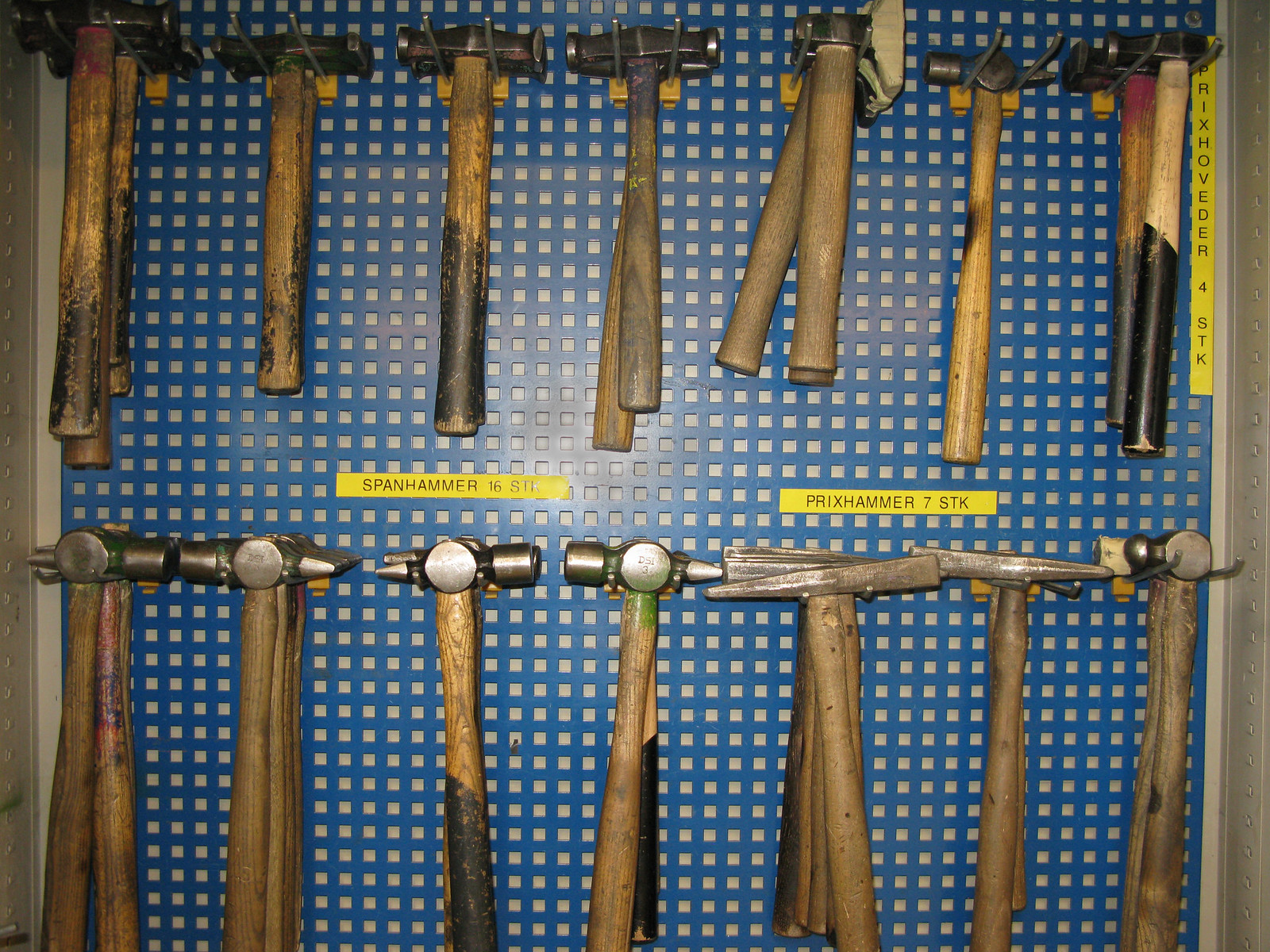The photograph showcases an array of hammers meticulously displayed on a blue grid-style pegboard. Each hammer is suspended from its head using metal prongs attached to wooden blocks, creating an organized and accessible arrangement. The hammers themselves vary widely in size, shape, and handle length. The majority have plain wooden handles, although some feature painted sections, notably black paint on the lower halves which is slightly worn on a few. The hammers also differ in head design; some have a flat head, others a spike, mallet-like heads, or double heads, contributing to a diverse collection.

Additionally, the pegboard includes two yellow labels with black text: on the right, the label reads "Prix Hammer 7 STK," and on the left, a similar label partially obscured by over-exposure, appears to say "Span Hammer 1-6.” Despite this variety, the hammers share a common utilitarian aesthetic against the structured backdrop of the blue mesh pegboard, emphasizing their readiness for use.